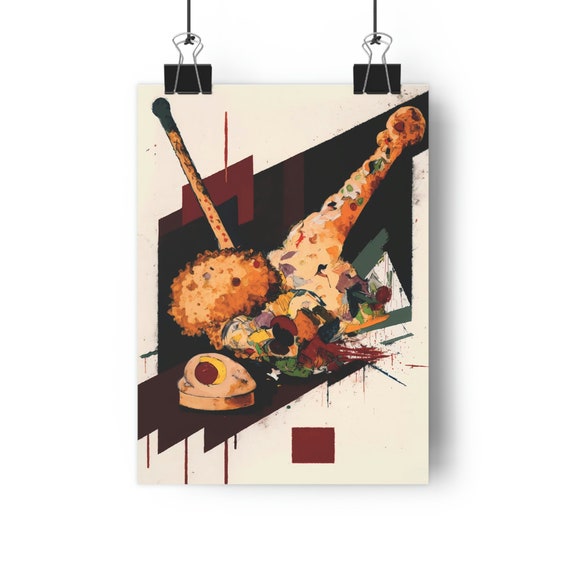This image appears to depict an abstract piece of artwork that is hung on a wall using two black binder clips, which have black strings attached to them for hanging. The poster has a beige or off-white background, with a prominent black trapezoidal shape occupying the center. This shape is intersected by loose geometric and interpretive forms and splashes of color. Noteworthy elements include a red L-shape and a square, a green and black oblong blob in the bottom left, a fuzzy yellow area in the upper left, and various other colors such as blue, yellow, and brown appearing in irregular shapes and splatters. There is what appears to be a depiction of food centered on the trapezoid, including a long chicken bone, what looks like a corn muffin top, and additional ambiguous food items. The combination of oxblood, black, green, red, shades of lilac, yellow, brown, and beige contribute to the vivid, almost chaotic composition on this canvas.